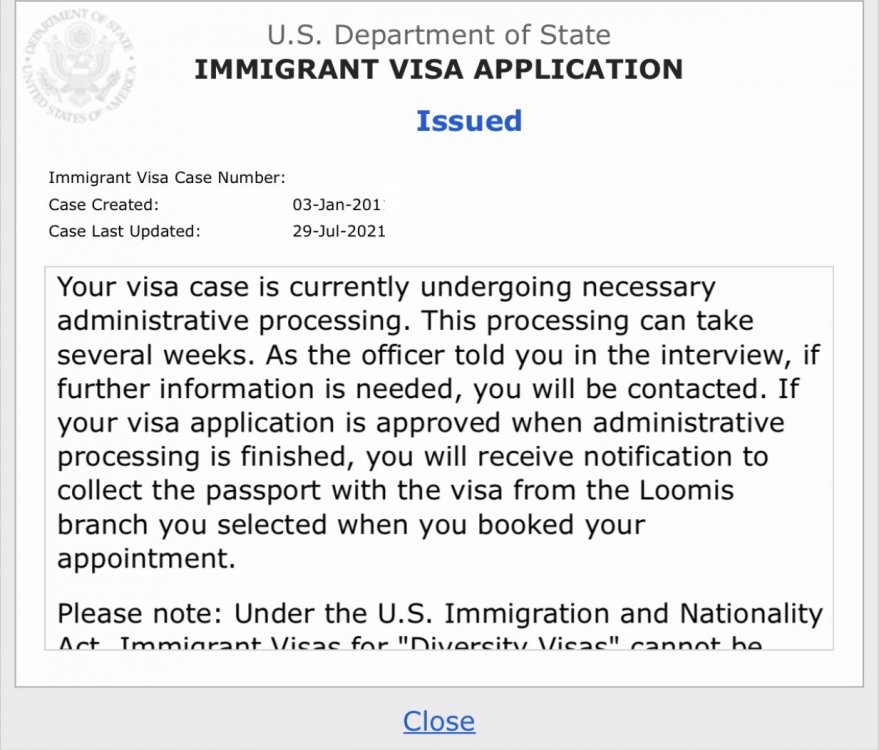The image shows an official immigrant visa application from the U.S. Department of State. In the upper left-hand corner, the document features a seal of the U.S. Department of State, signifying its authenticity. Below the seal, the text "U.S. Department of State" is clearly printed, and prominently, "IMMIGRANT VISA APPLICATION" is displayed in bold letters. The word "ISSUED" is printed in a bluish font, followed by a section labeled "Immigrant Visa Case Number," which is left blank.

Further down, the document indicates "Case Created" with the date "03-Jan-201," with the subsequent digits of the year obscured. It also states "Case Last Updated" with the date "29-July-2021." The text informs the applicant that their visa case is currently undergoing "necessary administrative processing," which may take several weeks. It mentions that if additional information is required, the applicant will be contacted as advised during their interview. The document ensures that upon approval of the visa, the applicant will be notified to collect their passport and visa from the Loomis branch selected during appointment booking. The text cuts off towards the end, and a “Close” button is visible at the bottom of the page.